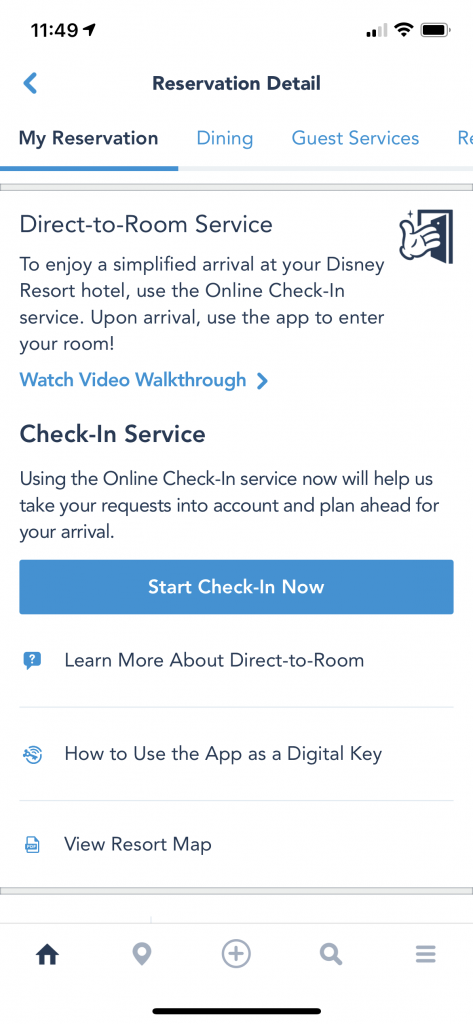Here's a cleaned-up and detailed caption for the image:

---

Screenshot of a cell phone displaying the reservation details page of a Disney Resort Hotel app. The top menu spans from left to right and includes sections labeled "My Reservation," "Dining," and "Guest Services." The "My Reservation" section is highlighted in black font with a blue bar underneath indicating it is currently selected. Directly below this section, there's an option titled "Direct-to-Room Service."

To the right, a large, cartoonish hand is shown opening a door to a room, with the hand appearing disproportionately larger than the door. Beneath the "Direct-to-Room Service" section, on the left side, text reads: "To enjoy a simplified arrival at your Disney Resort Hotel, use the online check-in service. Upon arrival, use the app to enter your room." Following this, a clickable link titled "Watch Video Walkthrough" is displayed with a forward arrow icon next to it.